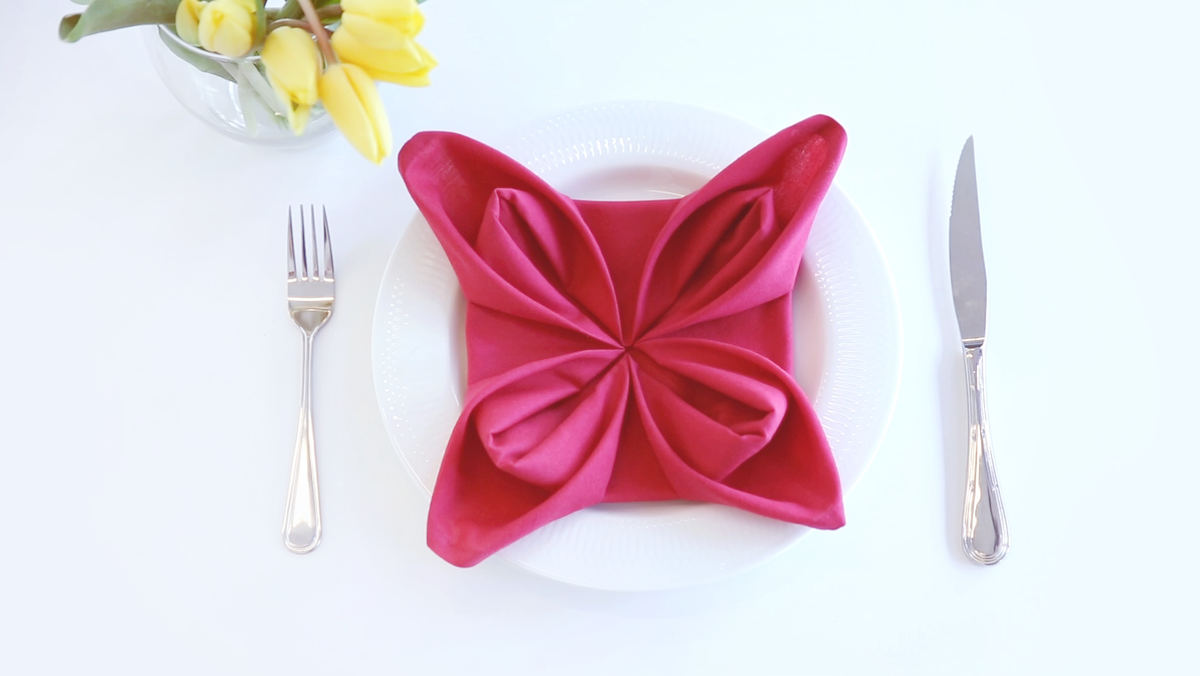The image portrays a meticulously arranged table setting, viewed from above. Central to this composition is a round white plate adorned with a fuchsia napkin intricately folded into a butterfly shape with four petal-like corners. To the right of the plate lies a silver knife with its blade turned inwards, and to the left, a matching silver fork. In the top left corner of the image, partially cropped, is a small glass vase holding freshly cut yellow tulips with visible green leaves. The entire setup rests on a pristine white tablecloth, emanating a formal and elegant atmosphere, reminiscent of a high-end restaurant or a sophisticated dinner party.